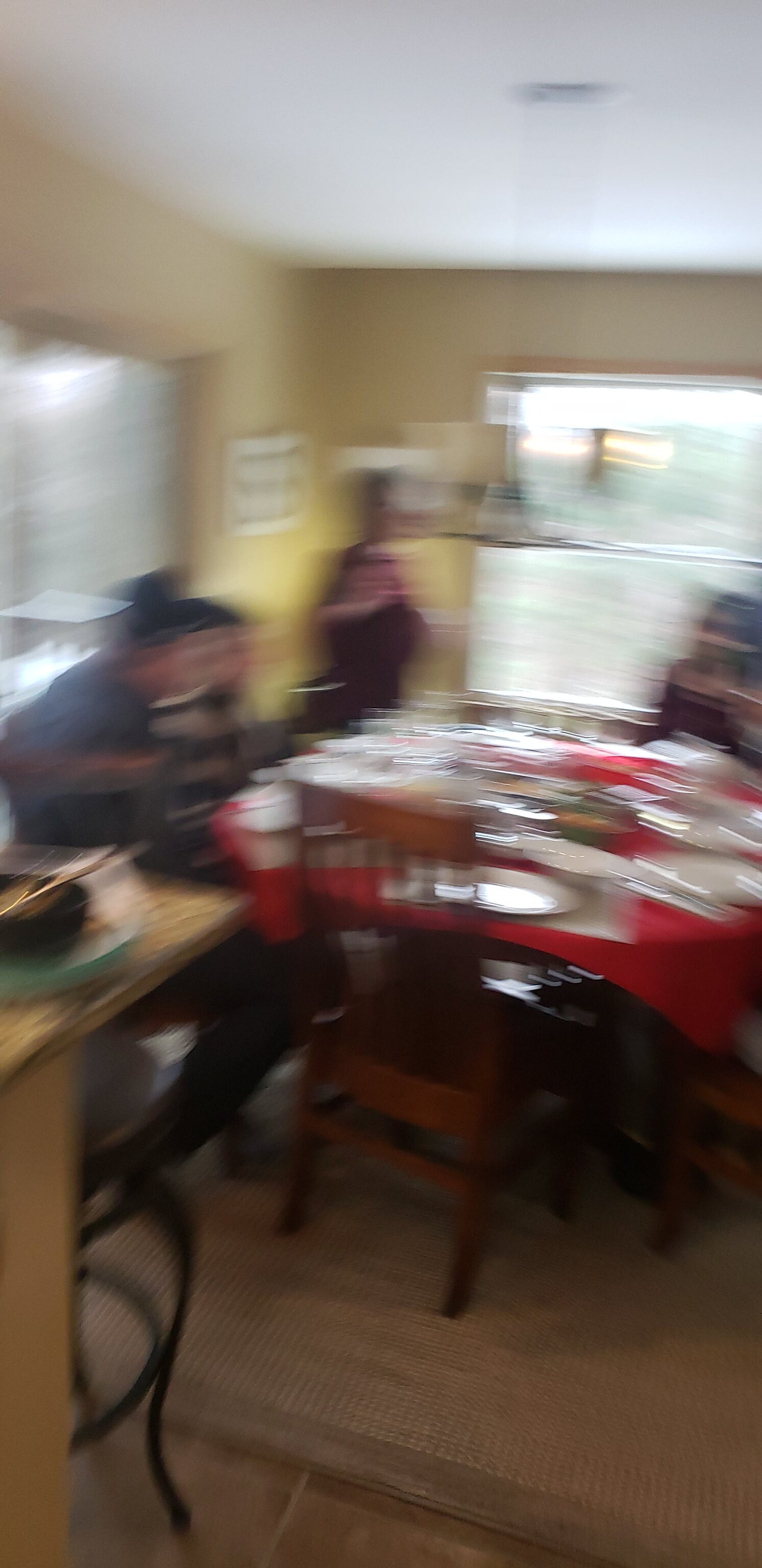This blurry indoor photograph, likely taken from a kitchen looking into a dining room, shows a well-lit scene featuring an oval dining table covered with a red tablecloth. The table is cluttered with numerous white plates and bowls, filling almost the entire surface. There are three to four indistinct figures seated around the table, their features obscured by motion blur, making it impossible to determine their age or gender. In the foreground, a wooden chair is slightly tilted to the left, suggesting it has been pulled out from the right. 

The background features a yellow wall with a large, square two-pane window that lets in natural light; the window lacks any curtains or shades. A low-hanging light fixture is positioned just above the table. To the left of the image, a corner of a yellow-painted counter with some dishes stacked on it is visible. The photograph is grainy and out of focus, and there are no words or text present in the image.